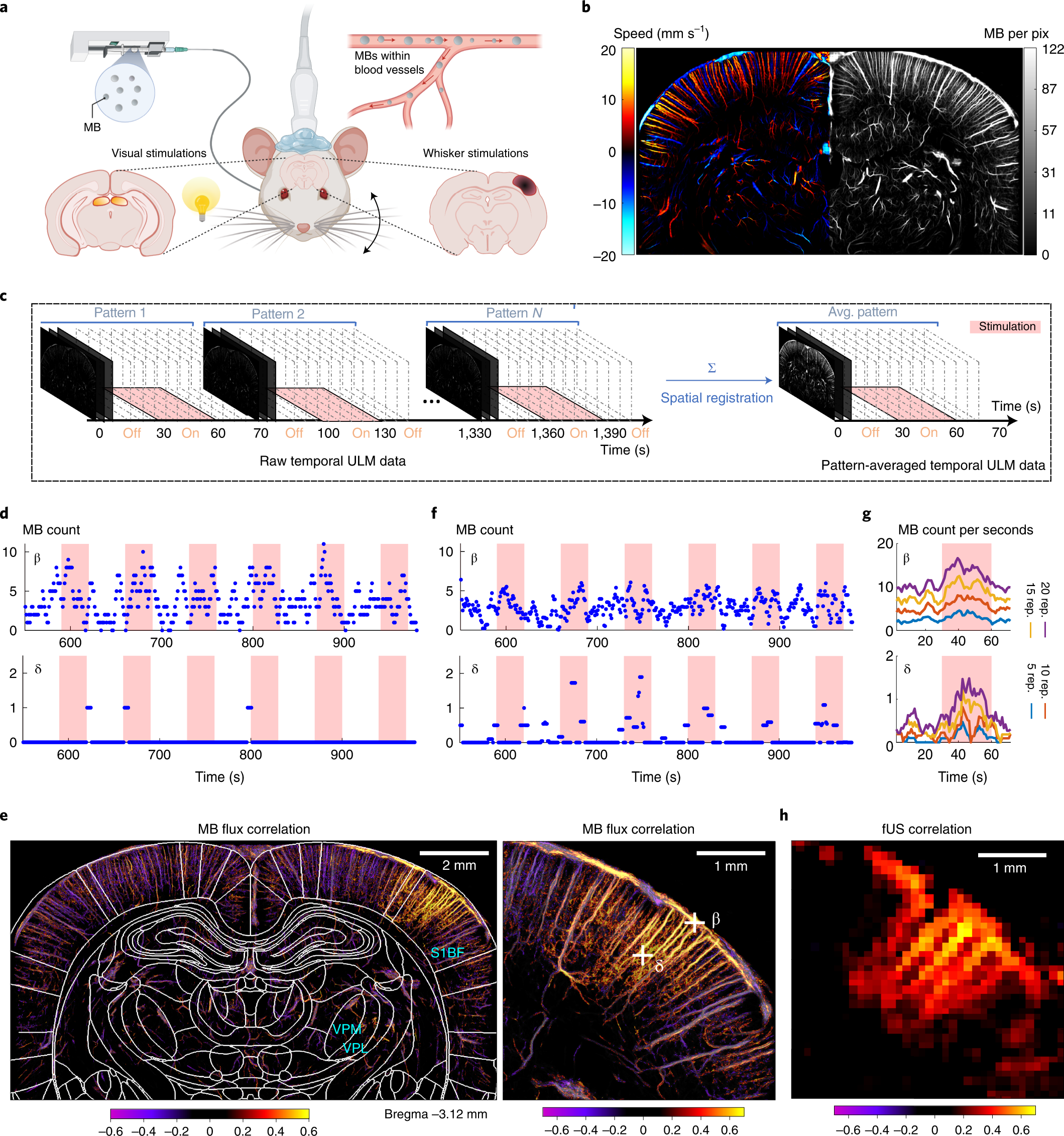The image presents a detailed scientific diagram set against a clean, white background. At the top center, there is an illustration depicting the face of a mouse or rat, characterized by white fur and pink ears. Moving to the lower left of the illustration, the text "visual stimulations to the mouse" is displayed, and adjacent to it on the right, it reads "whisker stimulations." 

Beneath these captions is a detailed chart labeled "raw temporal ULM data," featuring three distinct patterns labeled as Pattern 1, Pattern 2, and Pattern 3. In the upper right corner of the image, another chart is shown, which appears to measure speed with a scale ranging from 20 to -20 on the left side and 122 to 0 on the right. This part of the diagram might be related to the brain activity of the mouse or rat.

In the lower left corner, against a stark black background, there is what appears to be an x-ray image, potentially showcasing the internal structure or brain of the mouse or rat. The detailed and scientifically rich content of the image suggests it's aimed at elucidating neural responses to different types of stimulations in the animal subject.